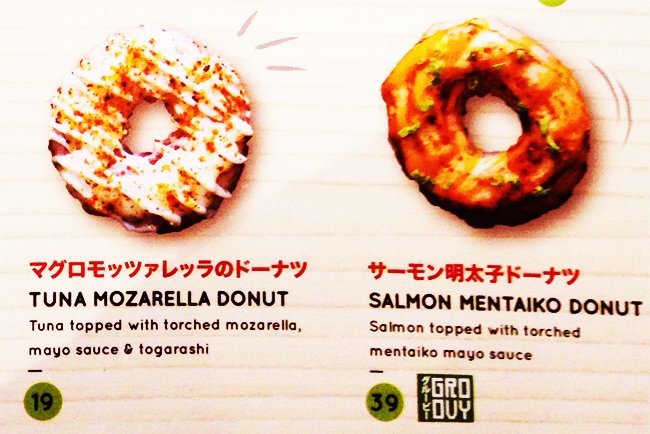The image depicts two creatively topped doughnuts placed on a light beige, softly-lined background with a subtle pink hue. The left doughnut is adorned with white, orange, and brown toppings, labeled "Tuna Mozzarella Doughnut." It features tuna crowned with torched mozzarella, a mayo sauce, and togarashi seasoning, and is marked with a green dot labeled "19." The right doughnut showcases orange, green-speckled, and brown toppings with areas of white, identified as the "Salmon Mentaiko Doughnut." This doughnut is topped with salmon and torched mentaiko mayo sauce, with a green dot labeled "39." Adjacent to the doughnuts, there's a square with the text "G-R-O-D-U-Y" in white lettering.